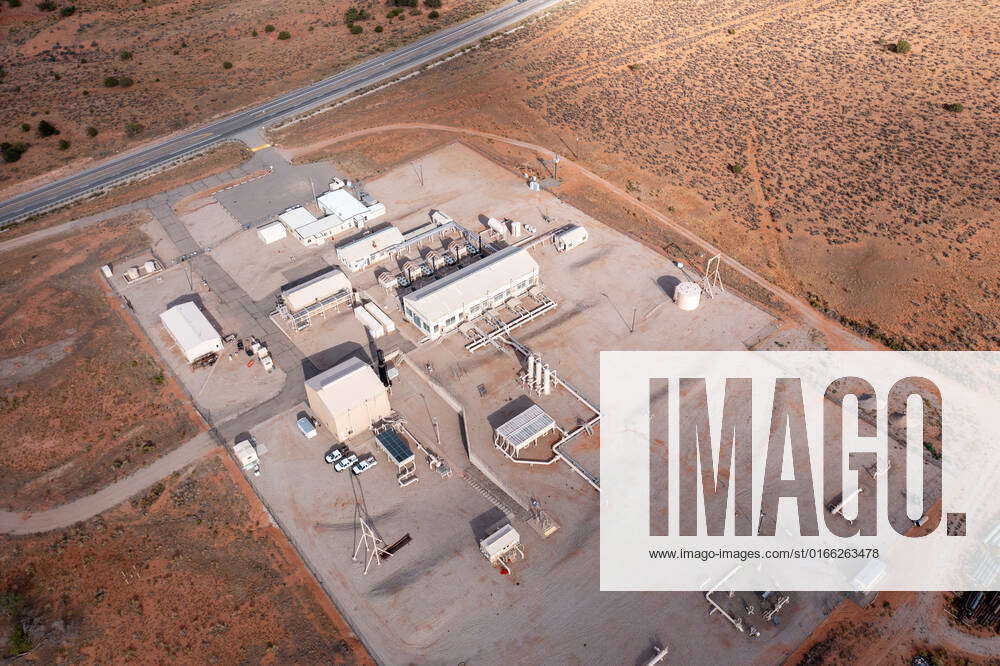An aerial, photorealistic image captures a factory-like assembly station situated in a barren, desert landscape characterized by sandy, reddish-orange clay with sporadic green shrubs. The focal point is a large concrete complex composed of numerous white buildings arranged in a rectangular layout, interconnected with piping. The complex features a parking lot with several vehicles, primarily trucks. In the image's upper left, a highway meanders from right to left, leading into a driveway that grants access to the industrial site. The bottom right corner prominently features a semi-transparent watermark with the text "IMAGO" above a web address, www.imago-images.com/st/0166263478. The photograph is taken during daylight, emphasizing the remote and industrial nature of the scene.